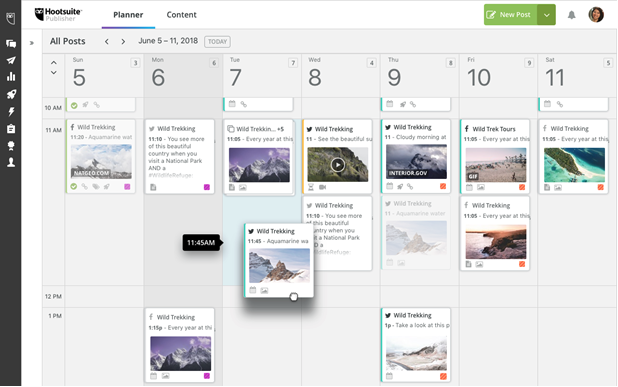The image depicts the interface of a calendar tool within the HootSuite Publisher program, featuring a clean white and gray design. On the left-hand side, there is a navigation pane with various icons, including text windows, a paper airplane, a graph, a rocket ship, a lightning bolt, a clipboard, and a person's head symbol. These icons likely represent different functionalities available within the program.

At the top of the interface, a toolbar displays the program’s name, HootSuite Publisher, emphasizing the current section, "Planner," which is highlighted. Another section labeled "Content" is also visible but not selected. On the far right of the toolbar, there is a green button labeled "New Post," followed by icons for alarms and the account owner’s profile.

Dominating the main section of the page is a calendar view covering the week from June 5 to June 11, 2018, laid out from Sunday to Saturday. Each day contains scheduled posts, with a recurring category titled "Wild Trekking" appearing on June 5 and June 7. The calendar entries include visual thumbnails of different scenes such as beaches and mountain ranges, indicating that the scheduled posts are related to various outdoor adventures and treks.

This detailed weekly planner showcases how the user has organized and scheduled their posts for the week, with specific activities and visual snippets planned and highlighted within the "Wild Trekking" theme.